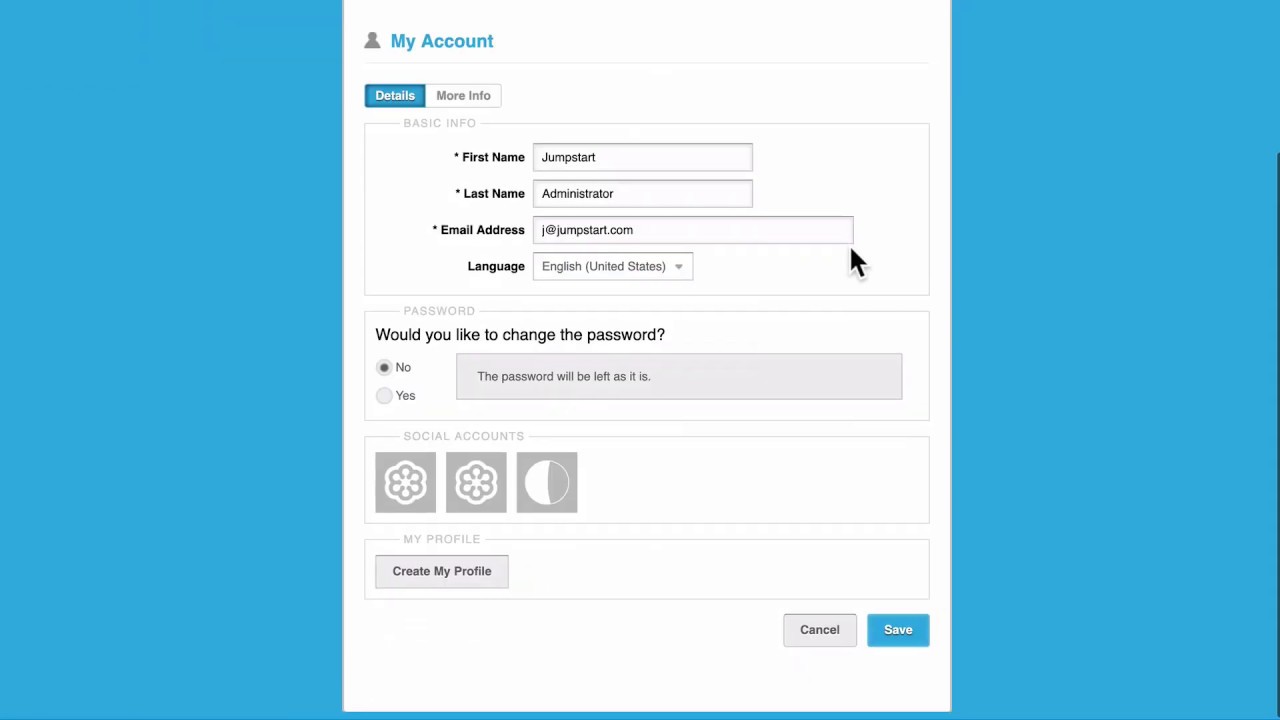The image showcases a user interface for a profile management page. The layout features a soft color palette, predominantly baby blue and white, with clean, delineated sections.

Starting from the left and right borders, there is a baby blue background that frames the central white space. Just beneath the baby blue borders, a thin blue line adds a subtle accent to the design. 

In the upper left-hand corner, a grey silhouette of a person symbolizes the user's account. Next to this icon, "My Account" is written in a baby blue font. Below it, there are two rectangular buttons: a baby blue button with white text labeled "Details," and a white button with grey text labeled "More Info."

In the center section, in very light grey font, the word "Baconshick Info" appears, though it may be slightly challenging to read due to its light color. Adjacent to it, the word "Black" appears, possibly indicating a heading. 

The "First Name" field follows, where the provided text "Jumpstart" is written in a white box. Beneath it, another heading "Last Name" is displayed in dark black text, and the user has entered "Administrator" in a corresponding white box, also in black font. 

Continuing downwards, there is a label marked "Email" in dark black text. The email provided appears in a white box with white text that says "J@Jumpstart.com."

The "Language" field is next, with a dropdown box displaying "English (United States)” in grey text. Below this, in very light grey, the word "Password" is printed.

Following this, the text "Would you like to change the password?" appears in black. Two radio buttons are placed on the left side: the first option says "No," and the second, directly below, says "Yes." If "No" is selected, a grey box with black text notifies the user that "the password will be left as is."

Toward the bottom, a heading titled "Social Accounts" is accompanied by small icons resembling two snowflakes and a crescent moon, possibly indicating different social media connections.

Lastly, options to manage the profile are available. "My Profile" and "Create My Profile" appear as clickable elements. The bottom section presents two buttons: "Cancel" and "Save," located at the bottom left and right corners, respectively, allowing the user to either discard changes or save them.